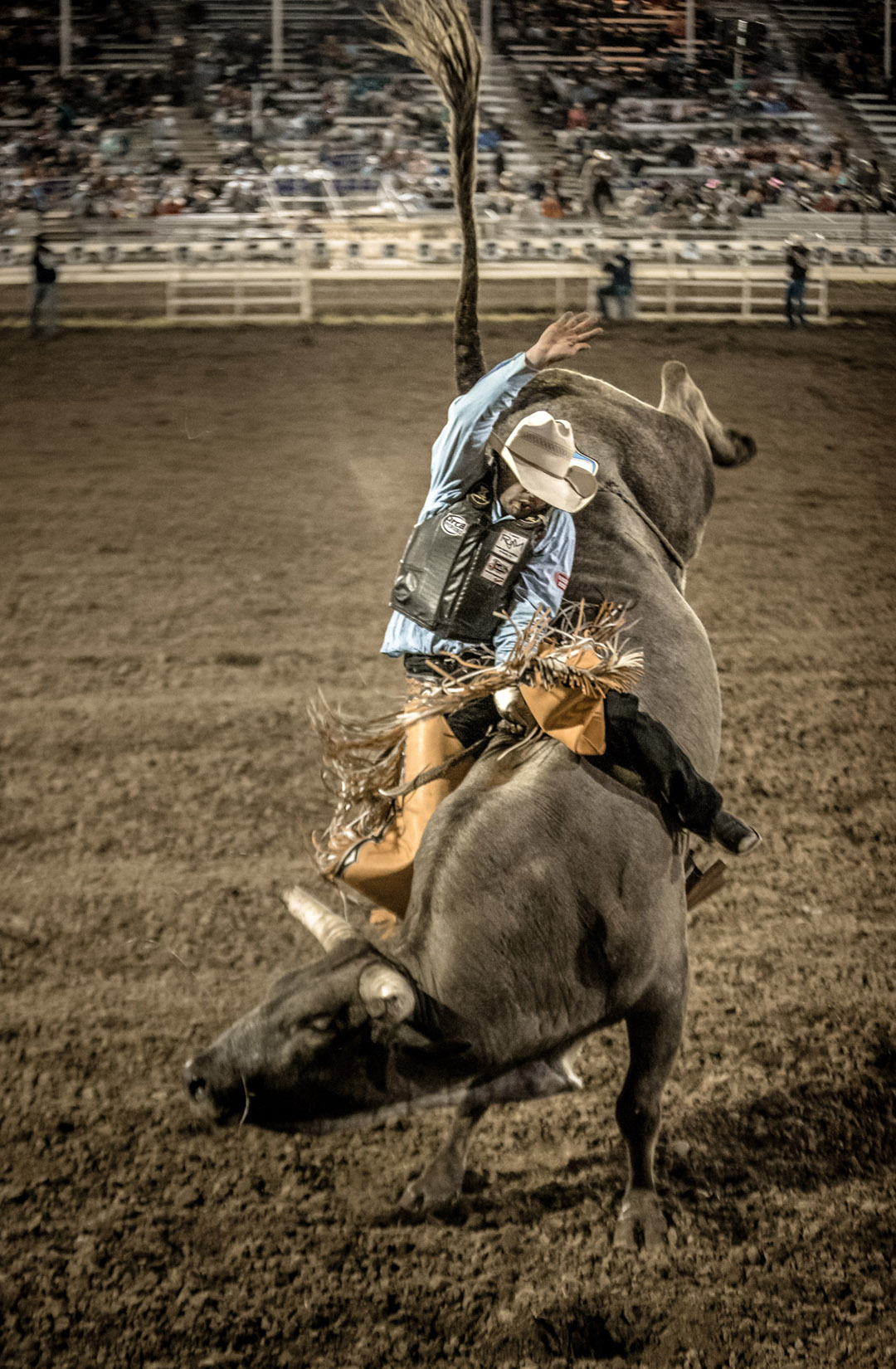In this high-quality image capturing the intense action of a rodeo scene, a cowboy is riding a bull in a field of brown dirt. The cowboy, sporting a white hat, a black protective leather vest, a light blue long-sleeve shirt, dark jeans, and tan chaps, is gripping the bull with his left hand while his right hand is raised in the traditional bull-riding stance. The bull, a dark gray beast, has its front legs planted firmly on the ground and its hind legs kicked high into the air, its tail pointing straight up in the ferocity of the moment. Behind them, the blurred background reveals large bleachers about 30% filled with a crowd, adding to the electrifying atmosphere of the rodeo. The clarity of the foreground contrasts with the indistinct figures of three individuals near a white gate, emphasizing the dramatic focus on the rider and bull engaged in this thrilling performance.